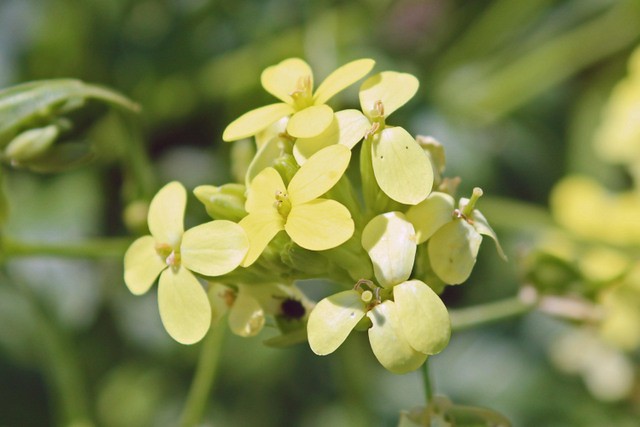This is an up-close color photograph showcasing a cluster of vibrant yellow flowers, each with four round, short petals reminiscent of hydrangeas. Central to each flower are small, similarly colored stamens. The cluster features approximately six flowers, though one flower on the right uniquely has only three petals. A tiny bee can be seen nestled among the blossoms. The background, rendered in greens and yellows, is blurred, indicating it is part of the same plant and suggesting a sunny day. The overall effect emphasizes the delicate beauty of the flowers against the softly out-of-focus foliage.